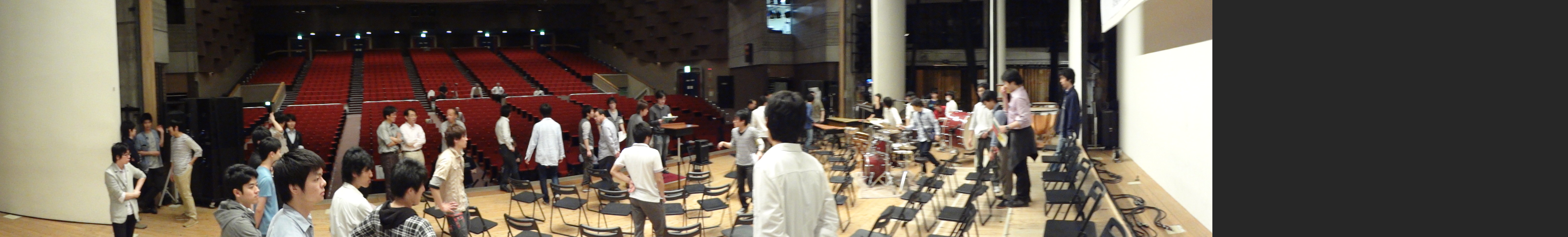The panoramic image captures the interior of a large theater or auditorium. The shot, taken from a distance, provides a wide-angle view of a well-organized venue. In the background, rows of red theater seats rise on an incline, arranged meticulously in aisles that extend towards the upper part of the photo. A hardwood stage, brightly lit, occupies the foreground where a group of about 30 to 40 people, mostly of Asian descent, are gathered. Most individuals are wearing white shirts and dark trousers, with one boy in a light blue shirt standing out on the left. The stage features several small black chairs, a drum kit, and is bordered by white walls on both the left and right sides. This setup suggests preparations for a music concert or similar event. On the right, beyond the white wall, a tall glass entryway is visible. Occupying the floor are also rows of metal folding chairs perpendicular to the theater seating, adding to the structured setup. Despite the numerous chairs and the bustling activity on stage, there is no audience present yet, indicating the event is likely in its preparatory phase.